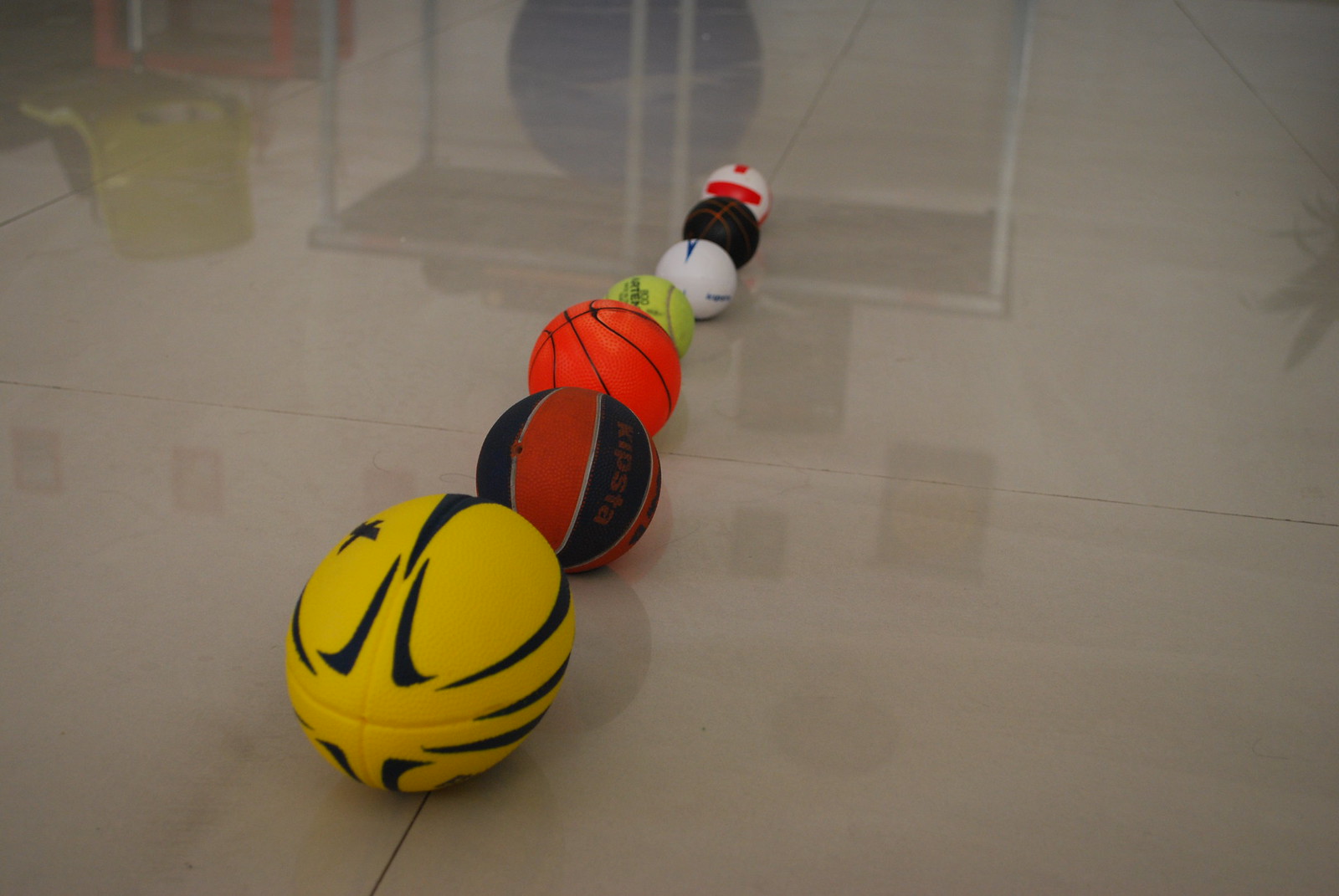The image showcases a highly polished, glossy gym floor, reflecting the surrounding environment, including a table or netting and a yellow chair. Arranged on a distinct, central black line are seven balls from various sports, organized from largest to smallest. The foremost ball is an oversized yellow and black football, significantly larger than a regular football. Following this is a red and black basketball with alternating colors. The third in line is a standard bright orange basketball. The fourth ball resembles a tennis ball but is two-thirds the size of the basketball. Next is a white ball with blue markings, succeeded by a smaller black and red ball, likely another type of tennis ball. The last in line is a red and white volleyball. The floor's surface is a sleek, brown concrete or similar material, enhancing the clarity of the reflections.